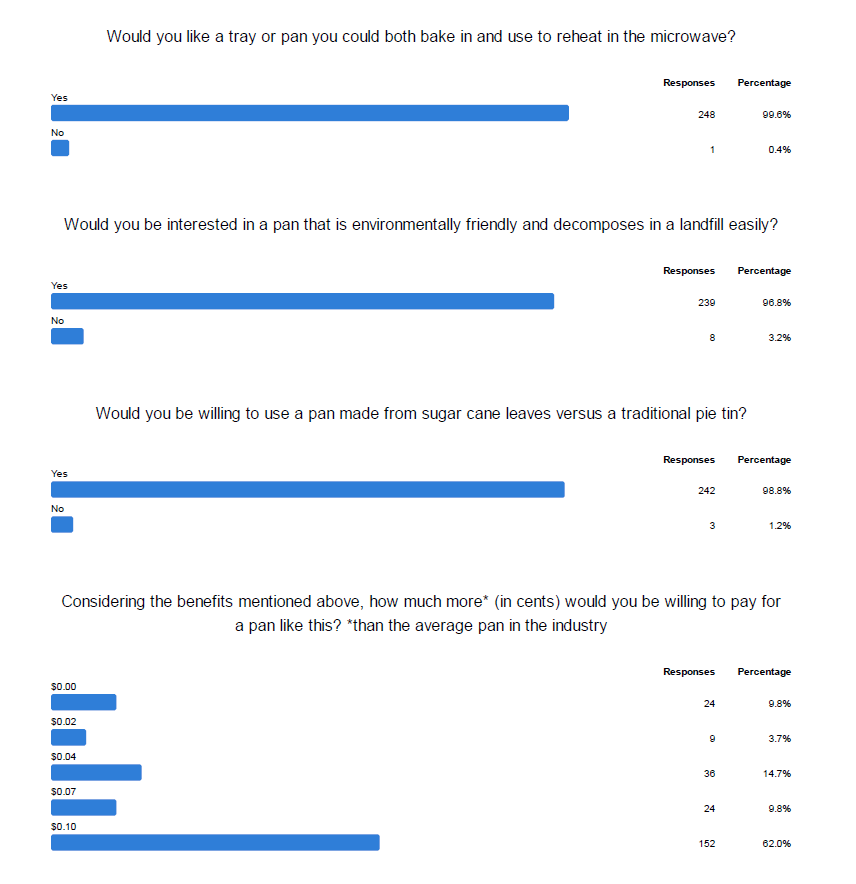This screenshot depicts the results of a survey regarding preferences for baking and reheating trays, with a focus on environmentally friendly options. 

The first question asks whether participants would like a tray or pan that can be both baked in and reheated in the microwave. The majority, accounting for 248 respondents (99.6%), answered "Yes," while only one person (0.4%) answered "No." Both responses are represented with blue bar graphs for visual comparison.

The second question inquires about interest in a pan that is environmentally friendly and decomposes easily in a landfill. Again, "Yes" is the predominant response with 229 people (96.6%) in favor, compared to 8 people (3.2%) who said "No."

The third question gauges willingness to use a pan made from sugar cane leaves versus a traditional pie tin. A significant majority, 242 participants (98.8%), support this option, while a small minority of 3 people (1.2%) are against it.

The final question addresses the price sensitivity of respondents regarding the environmentally friendly pan, asking how much more, in cents, they would be willing to pay compared to the average pan in the industry. The distribution of responses is as follows: 
- 24 respondents (9.8%) are not willing to pay any extra.
- 9 respondents (3.7%) would pay an additional two cents.
- 36 respondents (14.7%) are willing to pay an additional four cents.
- 24 respondents (9.8%) would pay an extra eight cents.
- 152 respondents (62%) are willing to pay an extra ten cents.

This detailed analysis highlights a strong preference for multifunctional and environmentally friendly baking and reheating solutions, with a notable willingness to pay a premium for such benefits.